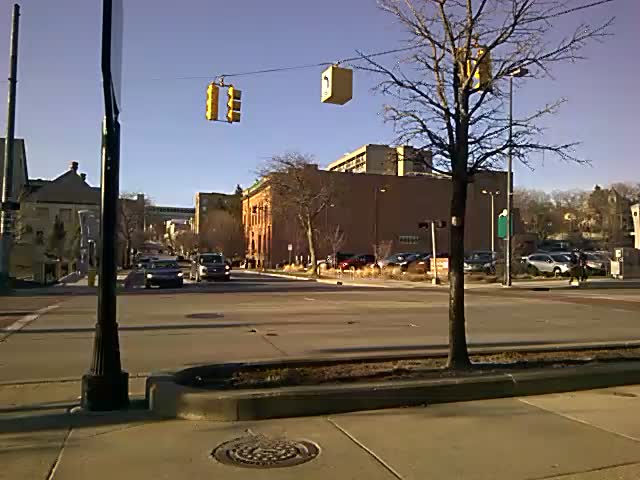The photograph captures a clear day at a T-shaped intersection in a downtown area, framed by a vivid blue sky. The image is taken from the top of the "T," slightly elevated from a sidewalk bordered by cement slabs and featuring a manhole cover. In the foreground, a leafless tree stands planted in a dirt area encircled by a cement outline. Close to it, a black light pole and a gray pole attached to a sign mark the left side of the sidewalk.

Facing the camera, two cars are at a stop sign, ready to proceed when the light changes. They are parked near a road that intersects horizontally, marked by traffic lights suspended above, with the one on the left glowing yellow. A white pedestrian crosswalk is visible on the far left. To the right, halfway up the image, a parking lot can be seen with several vehicles.

The backdrop features an array of small to medium-sized buildings, primarily brown and lighter brown with grayish roofs, all no more than a few stories high. The roads are gray, adding a subtle contrast to the overall scene.